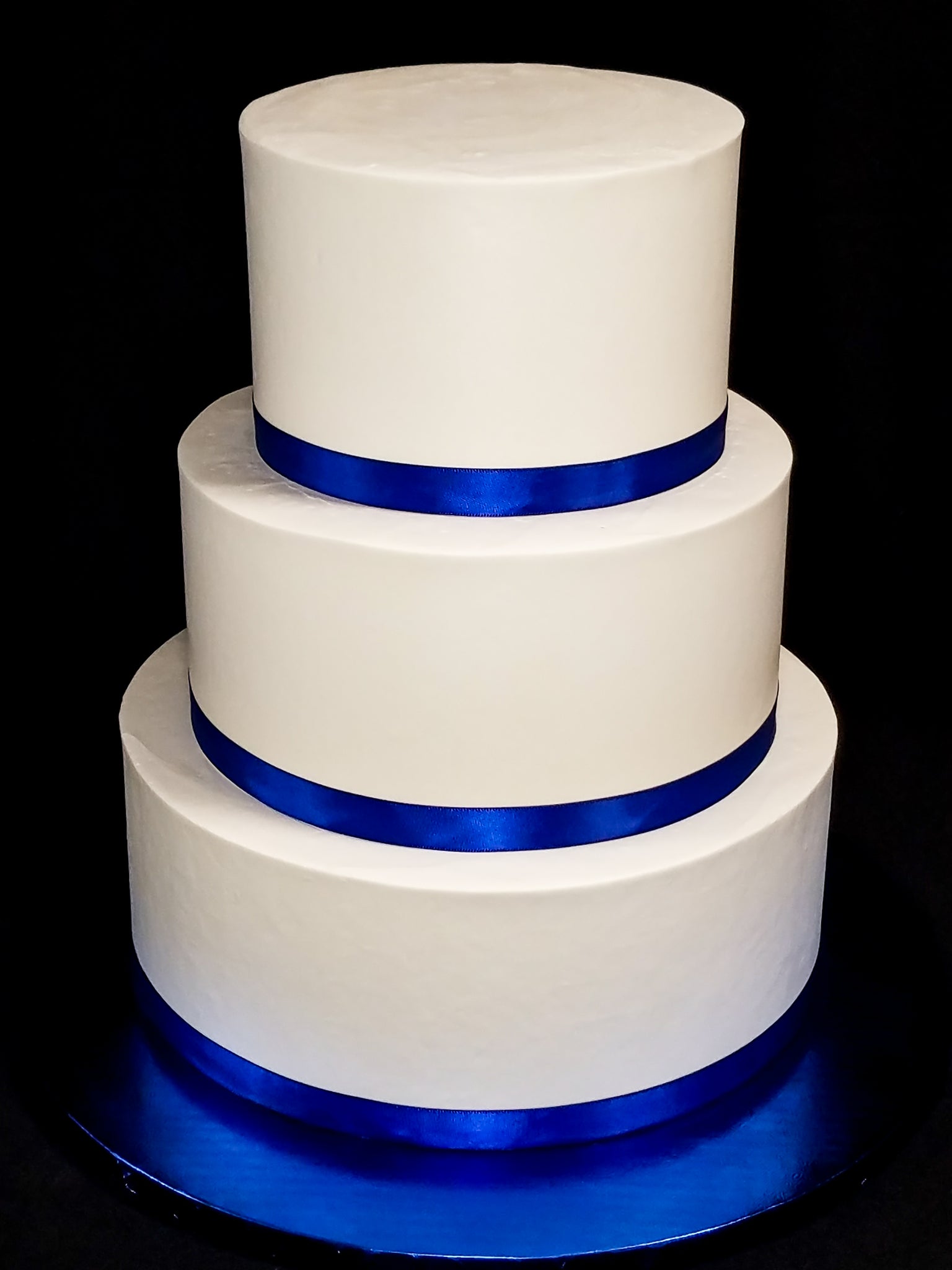The image is a vertically rectangular, two-tone photograph against a black background. It features a three-tiered, cake-shaped structure, with each tier wrapped at the bottom with a bright, shiny blue ribbon. The cakes, all in a pristine shade of white, are arranged from the largest tier at the base to the smallest on top. This stacked formation sits on a round blue base, further enhancing the vivid contrast against the dark backdrop. The photograph is borderless and devoid of any additional markings, focusing entirely on the elegant simplicity and striking color contrast of the tiered white cakes and their blue adornments.